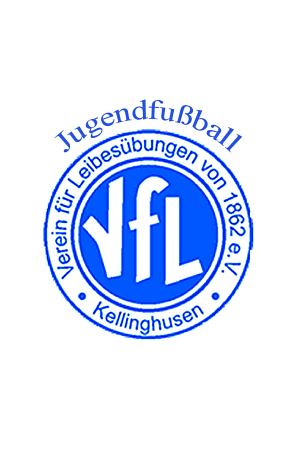The image showcases a detailed logo on a white background, primarily in blue and white colors. At the heart of the logo is a deep blue circle with the bold, white block letters "VFL" prominently displayed, where the "V" resembles a checkmark. Surrounding this central blue circle are two concentric blue rings containing German text. The text within these rings reads "Verein für Lebensbürgen von 1862 e.V." with "Kellinghusen" inscribed at the bottom. Above this circular logo, the name "Jugendfußball" is displayed in blue capital letters, indicating its association with a youth soccer team or league.